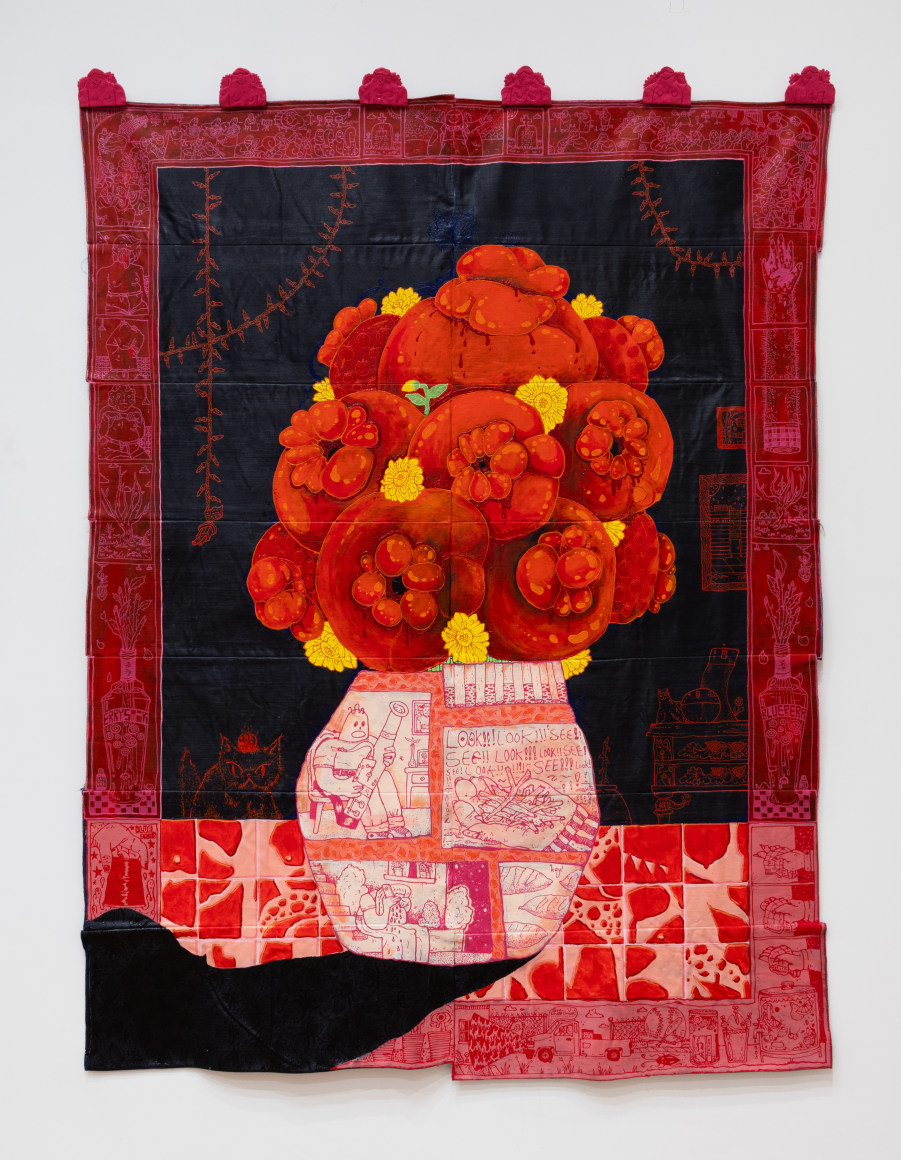This detailed image showcases a vibrant tapestry hanging vertically on an off-white wall. The tapestry is bordered by a bold red edge adorned with intricate white illustrations, including figures resembling tombstones, an angel, and clusters of people. The border transitions to a lighter red with images such as a pickup truck and a giant baseball at the bottom.

The central focus of the tapestry is a large, white vase filled with prominent red flowers and smaller orange and yellow blossoms. The flowers feature distinct circular or globular centers surrounded by petals, creating a striking visual contrast. The vase itself is elaborately decorated with multiple illustrations. Among the detailed depictions, there is a ghost-like figure holding a pipe, a hand clutching tree branches beneath text repeating "look, look, see, see", and a person with their head in their hands sitting on a bench in front of a house with stairs in the background. Additional images on the vase include a man holding a scroll, another structure, and possibly loaves of bread.

Behind the vase, the background is a mixed texture of red and light pink mosaic-like tiles. The upper two-thirds of the tapestry, inside the border, presents a black background with red drawings, including the image of a cat with a crown and shelves or paintings. This elaborate tapestry merges various artistic elements into a cohesive, yet intricately busy composition.